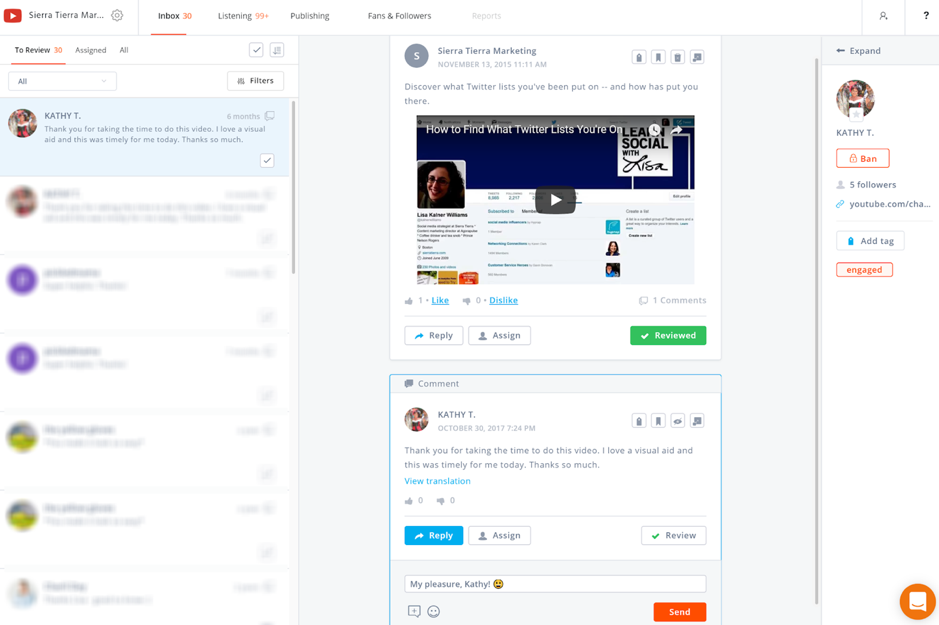The image depicts a detailed webpage layout for a popular website named "Era Trading Marketing." In the upper left corner of the webpage, there is a prominent red box featuring a white triangle pointing to the right. The top of the page displays several notifications in orange: "Inbox (30)" and "Listening (99+)," alongside sections labeled "Publishing," "Fans," and "Followers."

Beneath these sections, there is a category titled "To Review," which also has an orange bar and the number 30. Further filters labeled "Assigned" and "All" are available in this section. The first listed posting is from a user named Kathy T, who displays a profile picture. Her message, enclosed in a shaded blue box, reads, "Thank you for taking the time to do this video. I love a virtual, and this was timely for me today. Thanks so much!" Other user posts are visible but blurred out underneath Kathy’s message.

In the middle of the page, a box with the header "Discover what Twitter lists you've been put on and who put you there" offers guidance on determining which Twitter lists include the user. This section includes an image of Lisa—a woman with brown hair and glasses—alongside a video icon that suggests the presence of a watchable video content. 

Additionally, there's a "Reviewed" box in green located at the lower right corner. Kathy T's initial post appears again in a larger format with an option to reply. One reply is visible, marked with "My pleasure, Kathy."